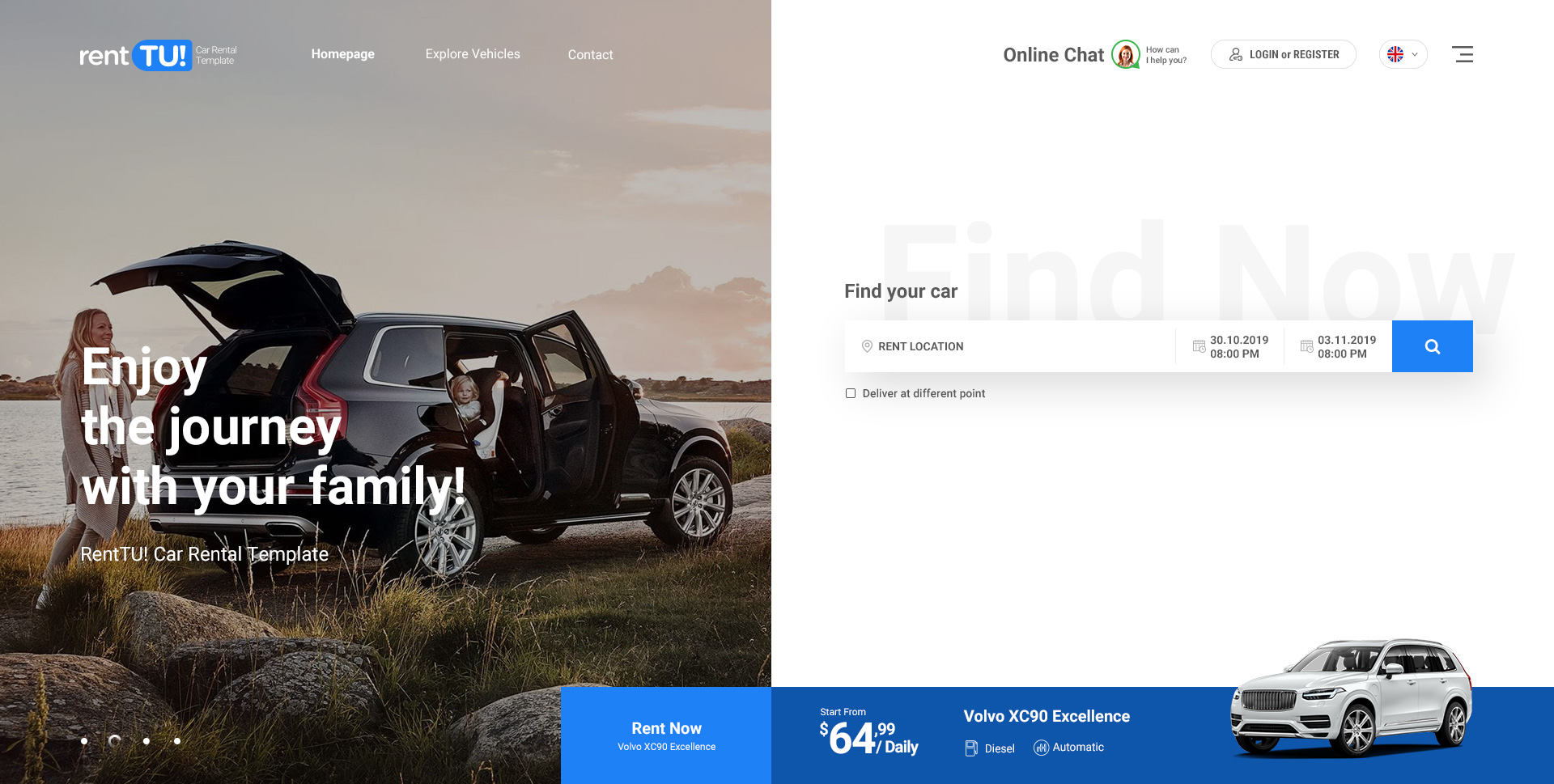A promotional image for a car rental company showcases a scenic outdoor setting. Featured on the left is a photograph of an SUV with its trunk and rear passenger door open. A smiling woman stands behind the vehicle, with a serene lake and majestic mountains in the background. In the foreground, patches of grass and rocks add to the natural beauty. Through the open passenger door, a child is visible in a rear-facing seat, highlighting the family-friendly aspect of the service. 

Across the top, the text reads, "Rent 2 Car Rental Template, Homepage, Explore Vehicles, Contact." In bold white letters, a headline states, "Enjoy the journey with your family, Rent 2 Car Rental Template." To the right, options for "Online Chat," "Login or Register" are present, alongside a prominent "Find Now" button and the prompt "Find Your Car." 

A dropdown menu offers "Rent Location" followed by rental dates and times, "30-10-2019, 8 pm" to "3-11-2019, 8 pm." Below, an image of a whitish-gray SUV is displayed with the model "Volvo XC90 Excellence." Pricing information indicates rentals "Start from $64.99 daily." Icons denote the vehicle features: "Diesel" fuel type and "Automatic" transmission, making the rental options clear and user-friendly.